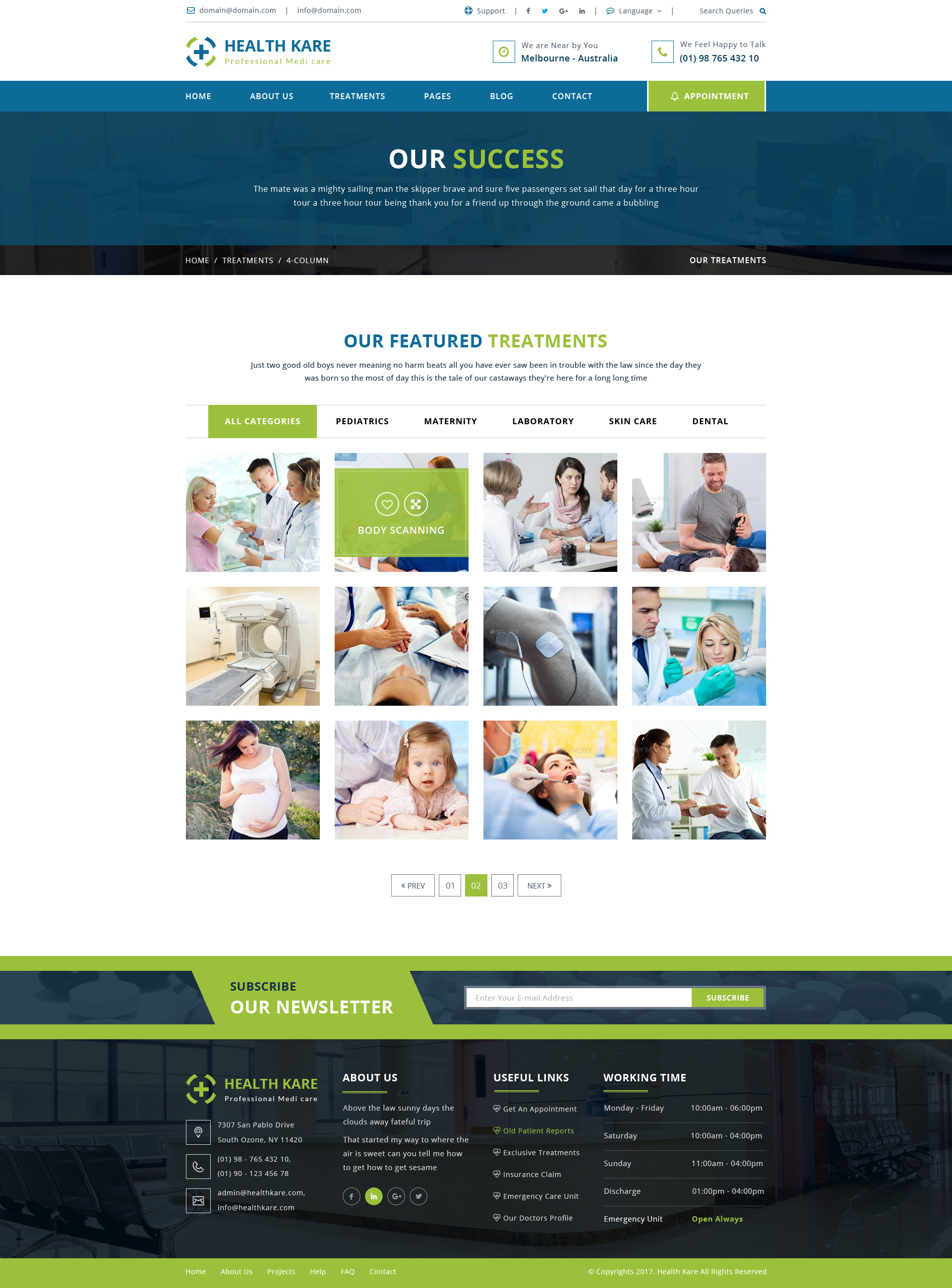The web page for "Health Kare" features a vibrant design and detailed layout. At the top, a bright blue banner spans the width of the page, displaying navigational options in white text: "Home," "About Us," "Treatments," "Pages," "Blog," "Contact," and in green text, "Appointment." These headings are situated on a crisp white background. In the upper left corner of the screen, the website's name, "Health Kare," is presented in dark blue text. Above this, there are icons for various social media platforms, offering ways to connect with Health Kare online.

Directly underneath the bright blue banner is a thicker navy blue ribbon with the phrase "Our Success" prominently displayed; "Our" is in white text, while "Success" is highlighted in green. Below this phrase is a line of tiny white text that is difficult to read. Following this is a thin black ribbon that stretches across the page, listing options: "Home," "Treatments," an unreadable word, and to the right, "Our Treatments."

The main section of the page features a white background with the heading "Our Featured Treatments." The phrase "Our Featured" is in blue, while "Treatments" is in green. Below this heading, users can select from different categories: "All Treatments," "Pediatrics," "Maternity," "Laboratory," "Skincare," and "Dental." The current selection is "All Categories," displaying 12 images in a grid format. These images depict various scenarios such as patients receiving different kinds of care, doctors consulting with patients, and medical equipment like an MRI machine.